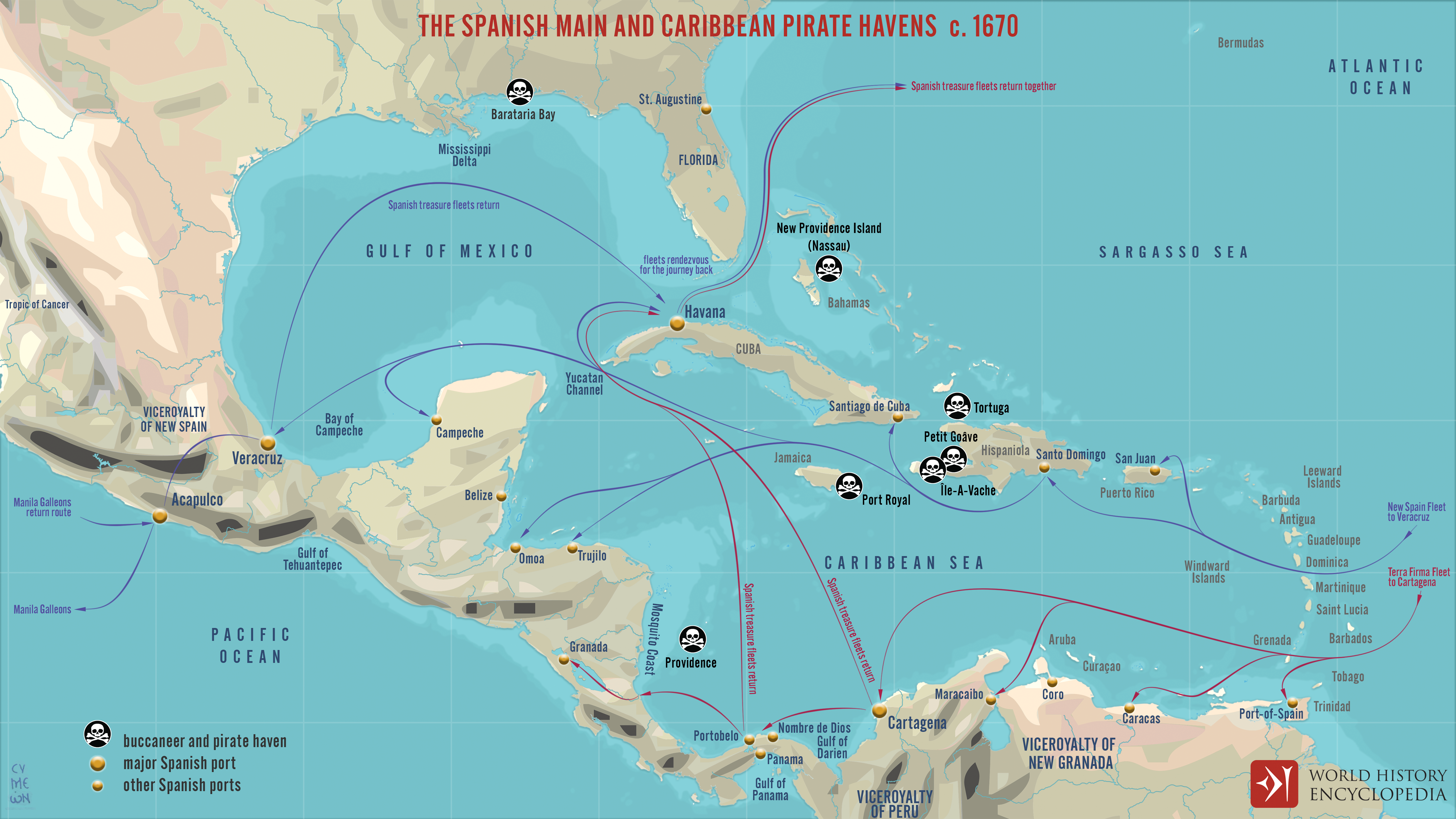This detailed map from the World History Encyclopedia titled "Spanish, Maine, and Caribbean Pirate Havens Circa 1670" vividly illustrates the geographical expanse of pirate activity during this era. It covers the southern United States, Mexico, and stretches down to the northern tip of South America. The map delineates major bodies of water, including the Pacific Ocean, Atlantic Ocean, Gulf of Mexico, Caribbean Sea, and the Sargasso Sea. Various states like Florida and prominent cities are labeled with blue and red circles, indicating important locations. Red and blue lines crisscross the map, tracing the routes traveled by pirates. The map marks major Spanish ports with larger dots, while smaller dots represent other significant ports. Notably, prominent pirate havens are highlighted, complete with a skull and crossbones symbol in the lower left corner, denoting buccaneer strongholds. The circled islands in the Caribbean and near the Mississippi Delta indicate areas frequented by pirate ships, reflecting the extensive network of waterways they navigated in the 17th century.